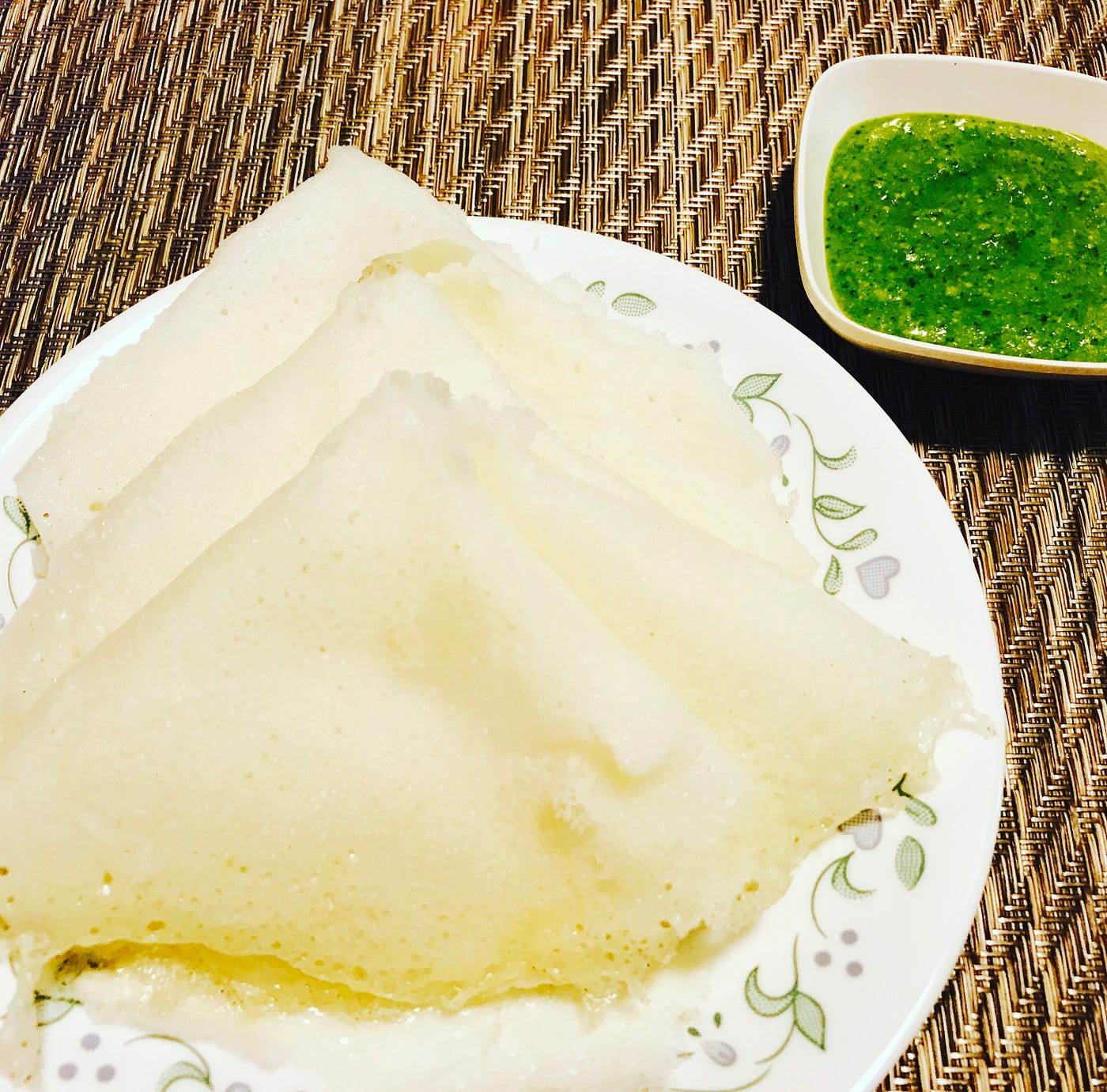This image captures a well-lit, top-angle view of an intricate food presentation, likely taken by a food blogger. The scene is set indoors, with a brown, tan, and white woven mat serving as the background. Centrally placed on the mat is a round, white plate adorned with subtle floral designs along its rim. On the plate rest three crispy, white, triangular flatbreads, possibly dosas or appams, common in Indian cuisine. Accompanying the flatbreads, situated in the upper right corner of the plate, is a small, square white bowl containing a vibrant green sauce or chutney. The meticulous details of the food and the care taken in presentation make this image eye-catching and appetizing.